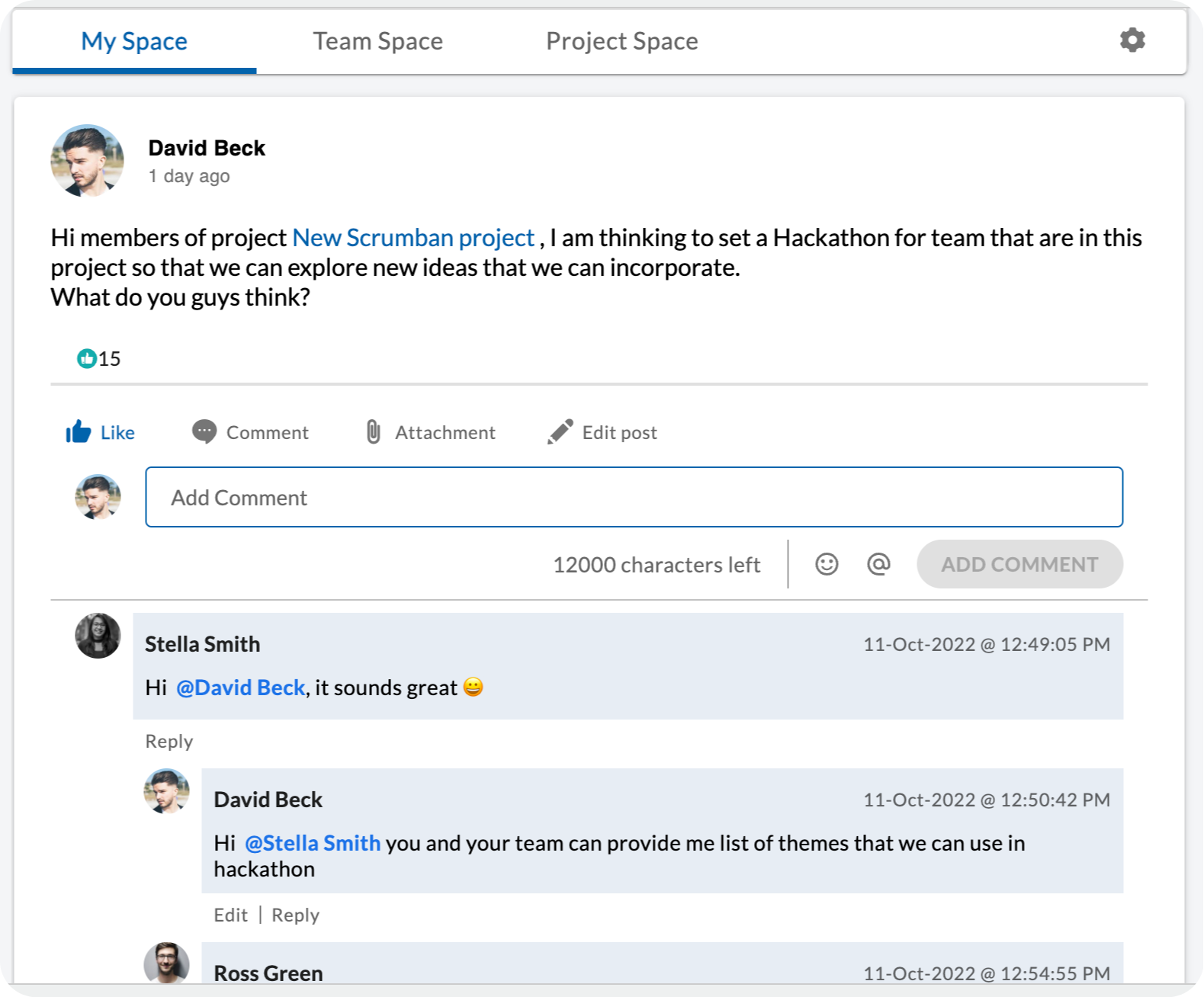The image displays an interface with a blue header at the top containing the titles "MySpace" on the left, "TeamSpace" next to it, and "ProjectSpace" further to the right. On the far right, there is a gear icon, likely for accessing settings. Below this header is a text box showing a profile picture of a man labeled "David Beck," who posted an update one day ago. The post reads: "Hi members of Project New Scrumping Project, I am thinking to set a hackathon for teams that are in this project so that we can explore new ideas that we can incorporate. What do you guys think?" The post has received 15 likes.

Beneath David Beck's post, there is a box labeled "Add a comment," which includes options for "Comment," "Attachment," "Edit Post," and a character count indicating there are 12,000 characters left.

A highlighted comment in a light blue box shows that "Stella Smith" responded on October 11, 2022, at 12:49:05 PM, saying: "Hi David Beck, it sounds great! 😊" David Beck then replied: "Hi Stella Smith, could you and your team provide me with a list of teams that we can involve in the hackathon?"